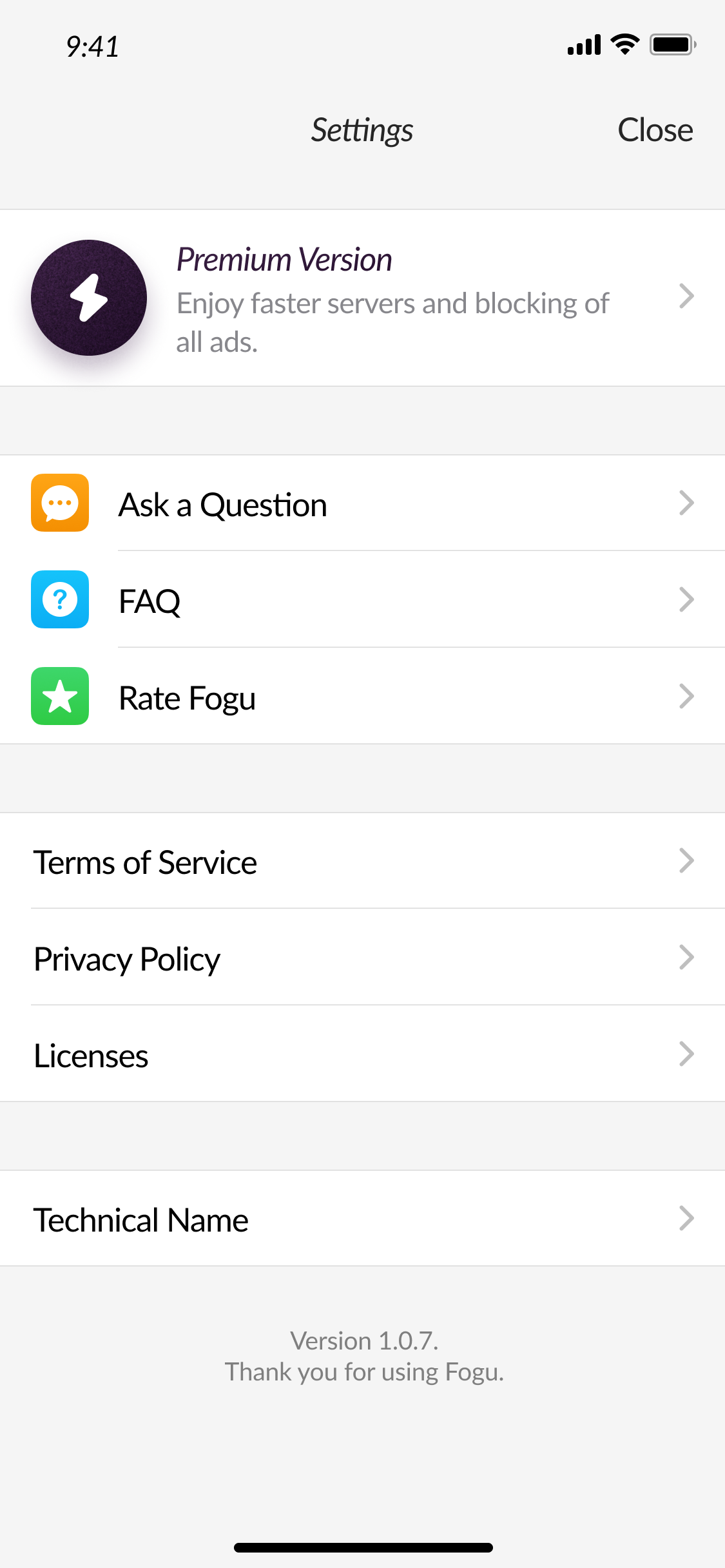The iPhone screenshot displays a settings page within an app called Fogu. In the upper left-hand corner, the time "9:41" is visible, while the upper right-hand corner shows a strong Wi-Fi connection with full signal bars and a fully charged battery icon. The settings page features a close button and a prominent section highlighting a premium version, characterized by a black circle with a white lightning bolt icon. This section offers benefits like faster service and ad-free usage, indicated by a right-facing arrow.

Further down, an orange icon with a speech bubble containing three dots prompts users to "ask a question" in black text. Below this, the frequently asked questions section is marked by an aqua bubble with a white circle and aqua question mark.

The next section invites users to rate the app with a white star inside a square, accompanied by the text "Rate Fogu." Following this are links to the Terms of Service, Privacy Policy, and Licenses, each with a gray right arrow to access submenus. At the very bottom, the screen displays a technical name coupled with another gray arrow to open a menu, along with the app version "1.07" and a message reading "Thank you for using Fogu."